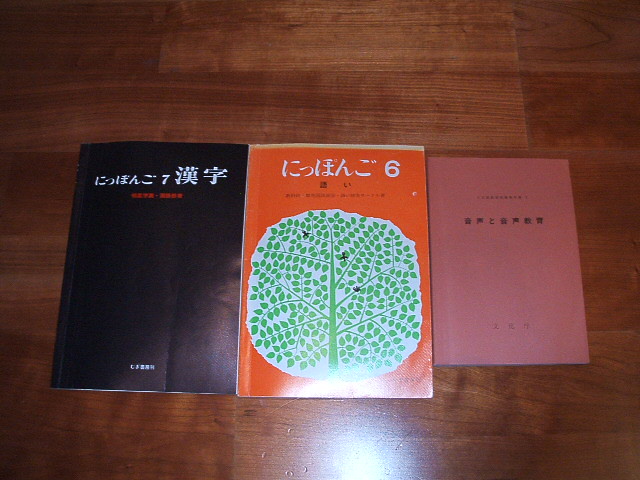The photograph captures a bird's-eye view of three books neatly arranged in the center of what appears to be a hardwood or laminate floor with a brown, board-like pattern. The background floor tiles reflect a subtle white light or flash at the bottom. The book on the left has a black cover adorned with white and red text, none of which is in English; it may be in an Asian language such as Japanese. The middle book is the same size as the first but features an orange cover with white and black text, also in a non-English script, and a whimsical, hand-drawn green tree with an abundance of leaves. Notably, the number six appears in white at the top right corner of this orange book. The third book, to the right, is slightly smaller and has a muted plum or pink cover with black text, also in a foreign script. The setting and photographic angle suggest the photo was taken from directly above, likely in a room with a wooden floor.